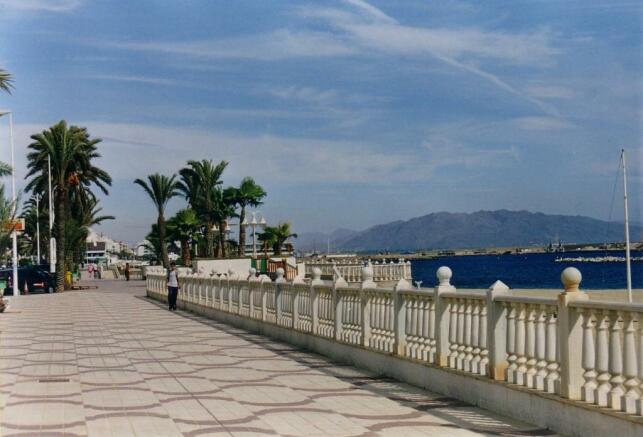The image captures a picturesque scene of a wide, patterned tile walkway stretching before a serene bay of water, set in a tropical climate. The walkway is composed of gray cement with distinctive darker gray sinusoidal lines and burgundy circular patterns. To the right, a white stone fence with decorative sculpted posts and curved wooden arms borders the path, providing a clear view of the deep blue water and the mast of a distant boat. A person can be seen walking near this fence. Palm trees with towering trunks and lush, drooping fronds frame the distant left side of the walkway. Farther right, across the ocean, a small mountain or large hill rises on the horizon under a bright blue sky dotted with soft white clouds, all illuminated by the daytime light.